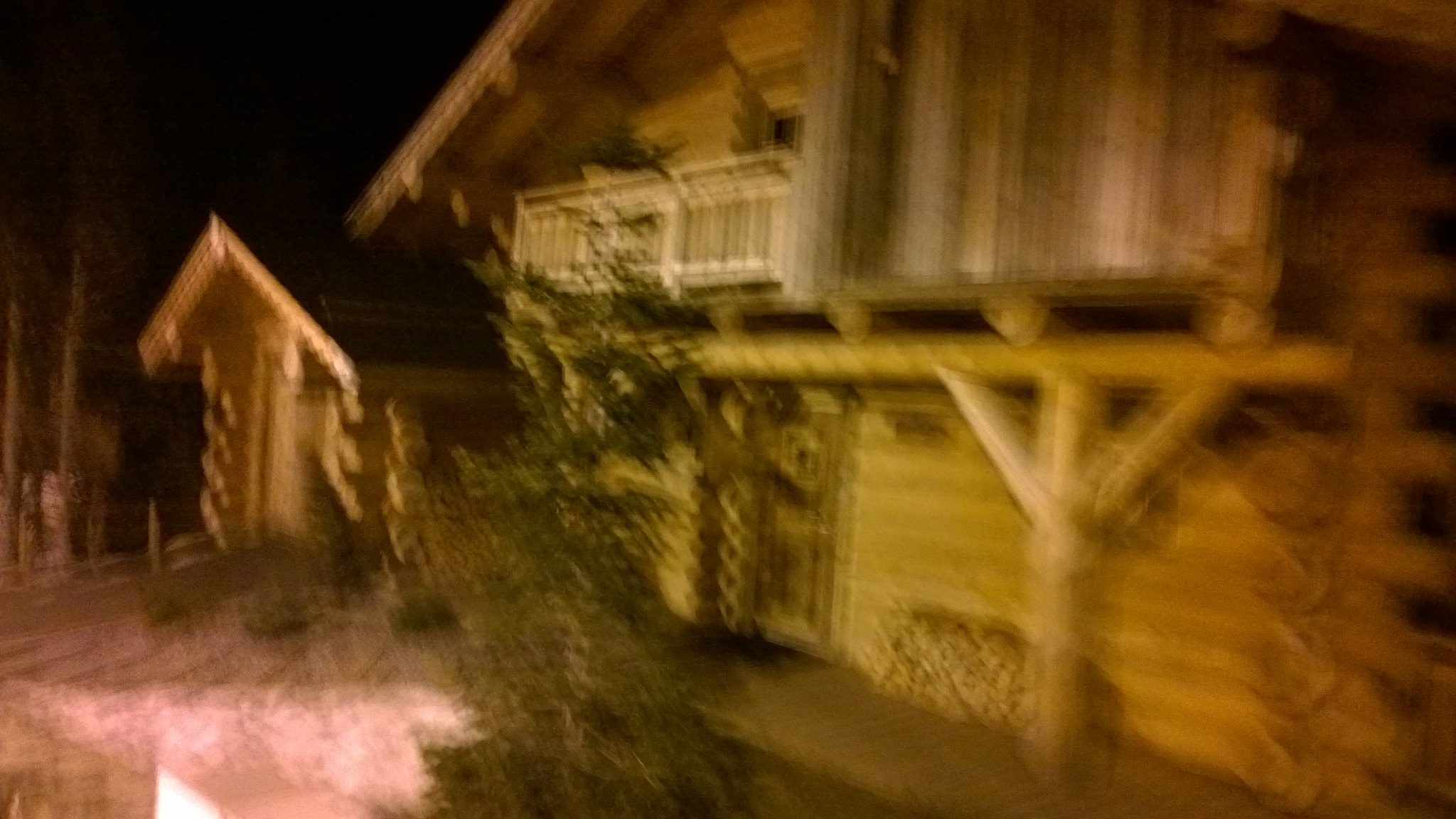This nighttime photograph showcases the exterior of a rustic log cabin surrounded by natural scenery. Despite the blurriness, you can make out the horizontally-arranged, medium-brown wooden boards that construct the cabin’s facade. To the left of the cabin stands another outbuilding, partially obscured by shadows.

A gravel driveway leads up to the cabin, adding to its rural charm. On the backside of the house, a door sits at ground level, with a rough-hewn pole extending upwards to support a vertical structure, possibly an outdoor shower.

A wooden balcony is situated to the left of this setup, with a window or door just behind it. Dominating the foreground is a large tree, its silhouette blending into the overall dark ambiance of the scene. The night sky is pitch black, devoid of stars, casting the entire image in muted tones of brown and green.